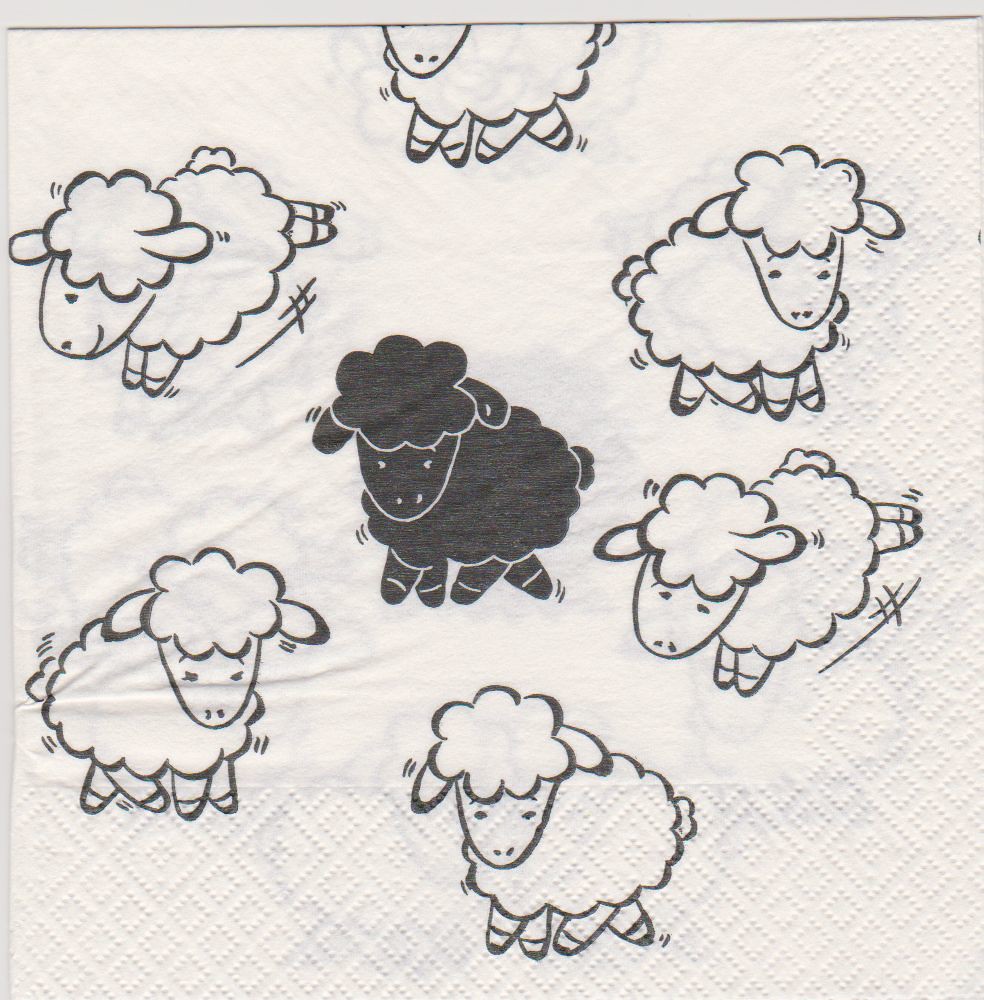Displayed on a slightly see-through white napkin is an artistic depiction of sheep, characterized by a textured bottom and right-hand edge with a diamond-shaped pattern. Six white sheep with furry outlines, drawn in black pen, encircle a single black sheep in the middle. The black sheep appears confused and scared, sitting on its hind legs with eyes indicative of fear. Little lines drawn around the sheep illustrate movement, suggesting that some of the white sheep are running while others are shaking. The black sheep’s solid color contrasts with the white, uncolored sheep. Behind the napkin, the same depiction is faintly visible due to the transparent quality of the fabric. Wrinkles are also noticeable on the cloth, adding a subtle texture to the image. The entire drawing takes up most of the composition, making the scene striking and expressive.